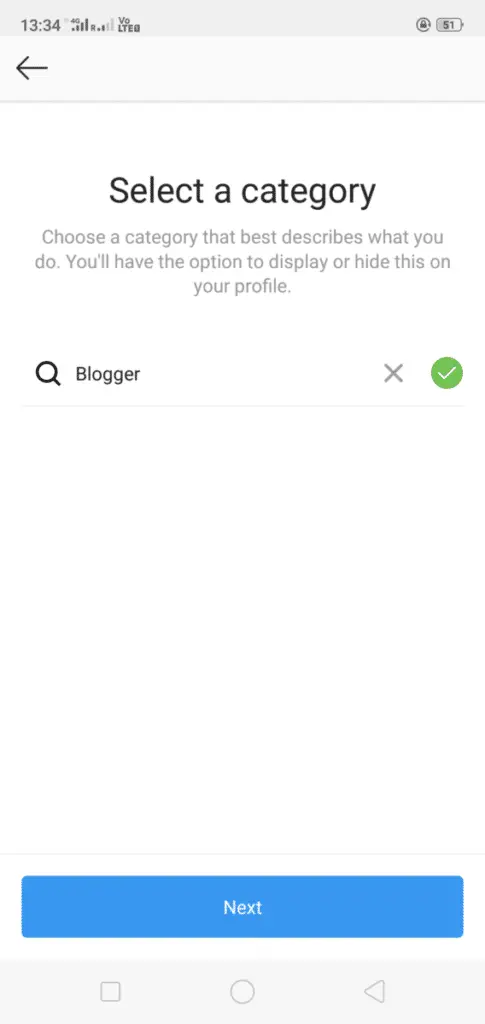This screenshot captures a minimalistic app page on a smartphone. At the top of the screen, a light grey header displays the time "13:34" on the top left, followed by five bars indicating 4G connectivity. Further right, another set of five bars shows LTE connectivity, with only the first two bars filled, while the remaining three are light grey. On the top right, a lock icon precedes a battery symbol showing half charge (51%).

Below this header is another light grey header featuring a black back arrow on the left. The main body of the screen is predominantly white, with the phrase "Select a category" in large black text centered at the top. Below this, a centered paragraph in smaller, light grey text advises, "Choose a category that best describes what you do. You'll have the option to display or hide this on your profile."

Further down, a text entry area is present with a black magnifying glass icon on the left. The word "Blogger," typed in black text with a capital "B," appears to the right of the icon. Adjacent to this on the right edge of the box are a light grey "X" and a green circle bearing a white checkmark. The screen then features a large expanse of empty white space, interrupted only by a thin grey line at the bottom.

Near the bottom of the screen, a medium blue rectangle with rounded corners displays the word "Next" in small white text centered within it. Finally, at the very bottom, a light grey box houses three icons: a rounded square on the left, a circle in the center, and an equilateral triangle on the right, with one point facing left, another up, and the third down.